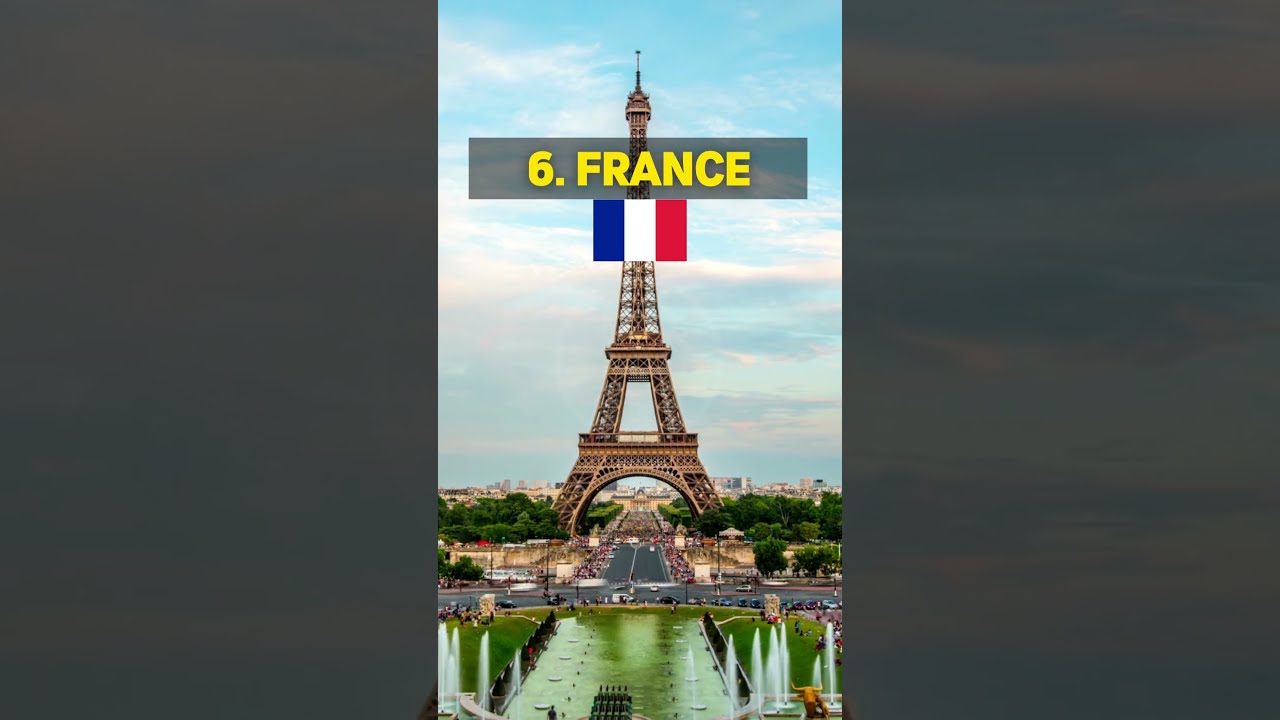This image prominently features the Eiffel Tower positioned in the left and right thirds, with a dark background. Over the Eiffel Tower near the top, there's a narrow gray strip with the yellow text "6th period France." Just below this text is the French flag, displaying the blue, white, and red colors.

The Eiffel Tower itself, depicted in a bronze hue, stands tall, extending slightly past the center of the image. The sky behind it is a serene light blue with scattered white clouds. At the base of the tower, a verdant grass field is visible, flanked on either side by lush green trees. The surrounding area shows a bustling scene with many people, streets, and cars.

Further down, before reaching the foreground, a rectangular reflecting pool with greenish water is present. The pool is divided, hinting at multiple sections. Additionally, small fountains on either side of the pool shoot up streams of white water, adding a dynamic element to the scene. The background stretches out into the cityscape, where more people, buildings, and streets can be seen, seamlessly blending into the horizon.